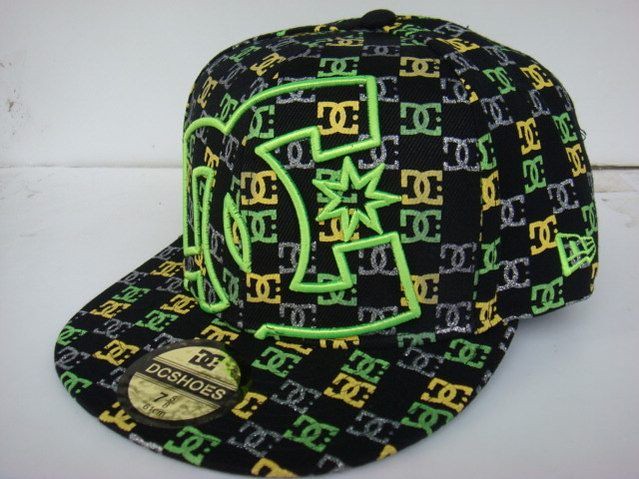This image is a vibrant, detailed product photograph of a DC brand ball cap, presented in landscape orientation against a clean, white background that could be a countertop or a wooden table. The hat itself is predominantly black, adorned with a pattern of the DC logo in neon green, yellow, and purple across the entire surface. Prominently featured on the front of the cap is a large lime green DC logo with a star symbol inside the letter "C." Additionally, the brim of the cap showcases a circular medallion design in off-white, containing a black horizontal bar that reads "DC Shoes" in white lettering, along with "size 7" in black text. The style of the image is characterized by representational realism, emphasizing the product details meticulously.